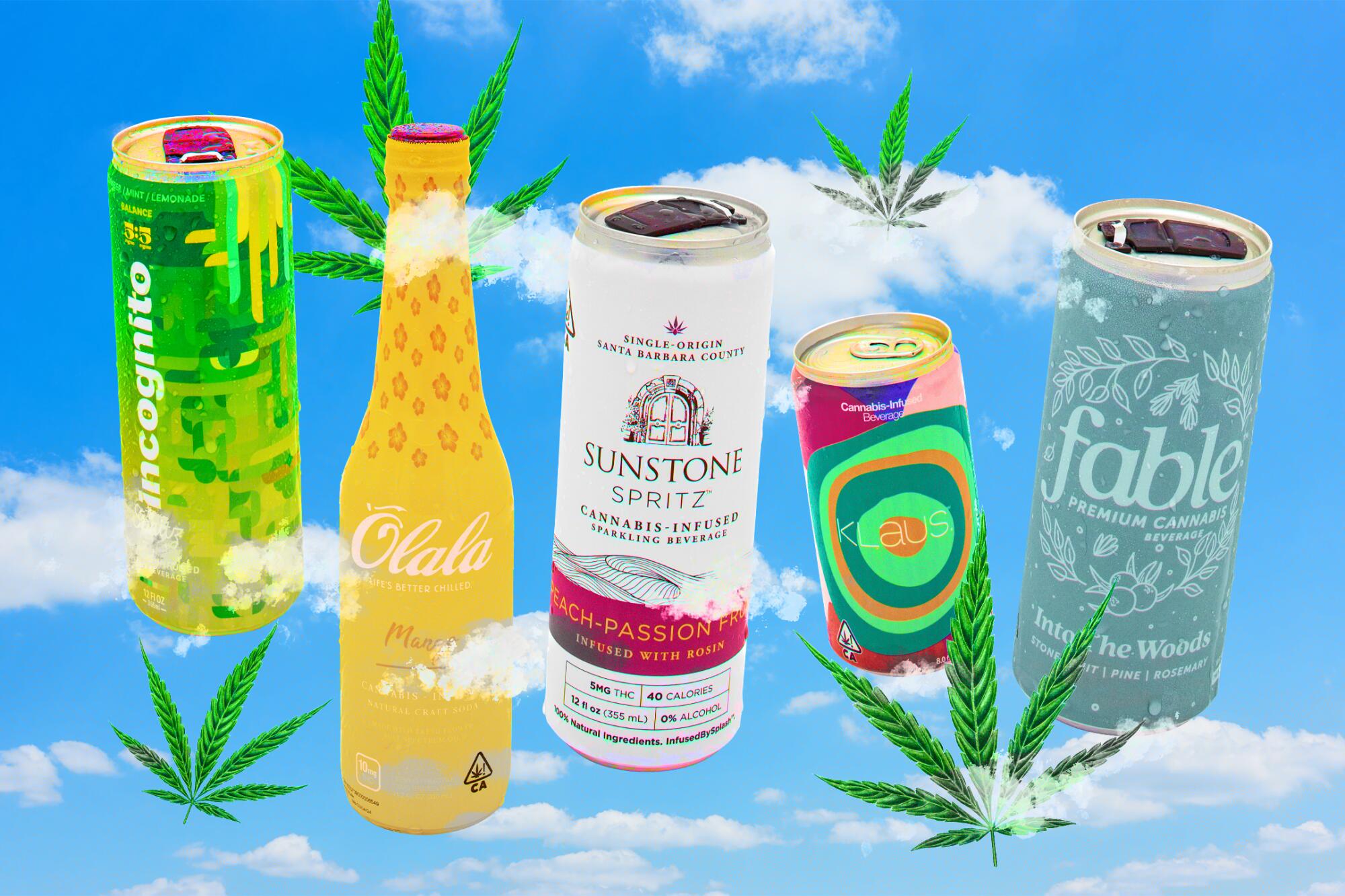The image is a vibrant, multi-color digital piece that serves as a promotional advertisement. It features a horizontally rectangular layout set against a vivid blue sky adorned with fluffy white clouds. Interspersed throughout the image are four marijuana leaves of varying sizes, adding to the cannabis-themed design. The background lacks a border, allowing the scene to flow seamlessly.

Central to the image are five different cannabis-infused drink containers, each distinct in its appearance and branding. From left to right:

1. **Incognito**: A tall, digital-green aluminum can with abstract gold patterning and a pop-top lid. The design features simple white horizontal and vertical lines, emphasizing the 'incognito' nature of the brand.

2. **Oh Lala**: An elegant, orange bottle with a long neck, adorned with a floral pattern and the words "Oh Lala" in decorative script. The bottle suggests a mango flavor and is also cannabis-infused.

3. **Sunstone Spritz**: A sophisticated white aluminum can with a black tab, prominently displaying "Single Origin Santa Barbara County." The label mentions it is infused with peach and passion fruit flavors and includes details such as 5 milligrams of THC, 40 calories, and 0% alcohol.

4. **Klaus**: A visually dynamic can with a green and orange motif. The design is described as a swirling cyclone of colors including pink, purple, and cobalt blue. It carries a bold, poppable top.

5. **Fable Premium Cannabis**: A gray aluminum can styled in an old-fashioned font, reading "Fable" with the subtitle "Into the Woods." The design includes imagery of berries and leaves arranged like a wreath.

The drinks are neatly arrayed across the center of the image, providing an organized yet lively display that captures the viewer's attention.